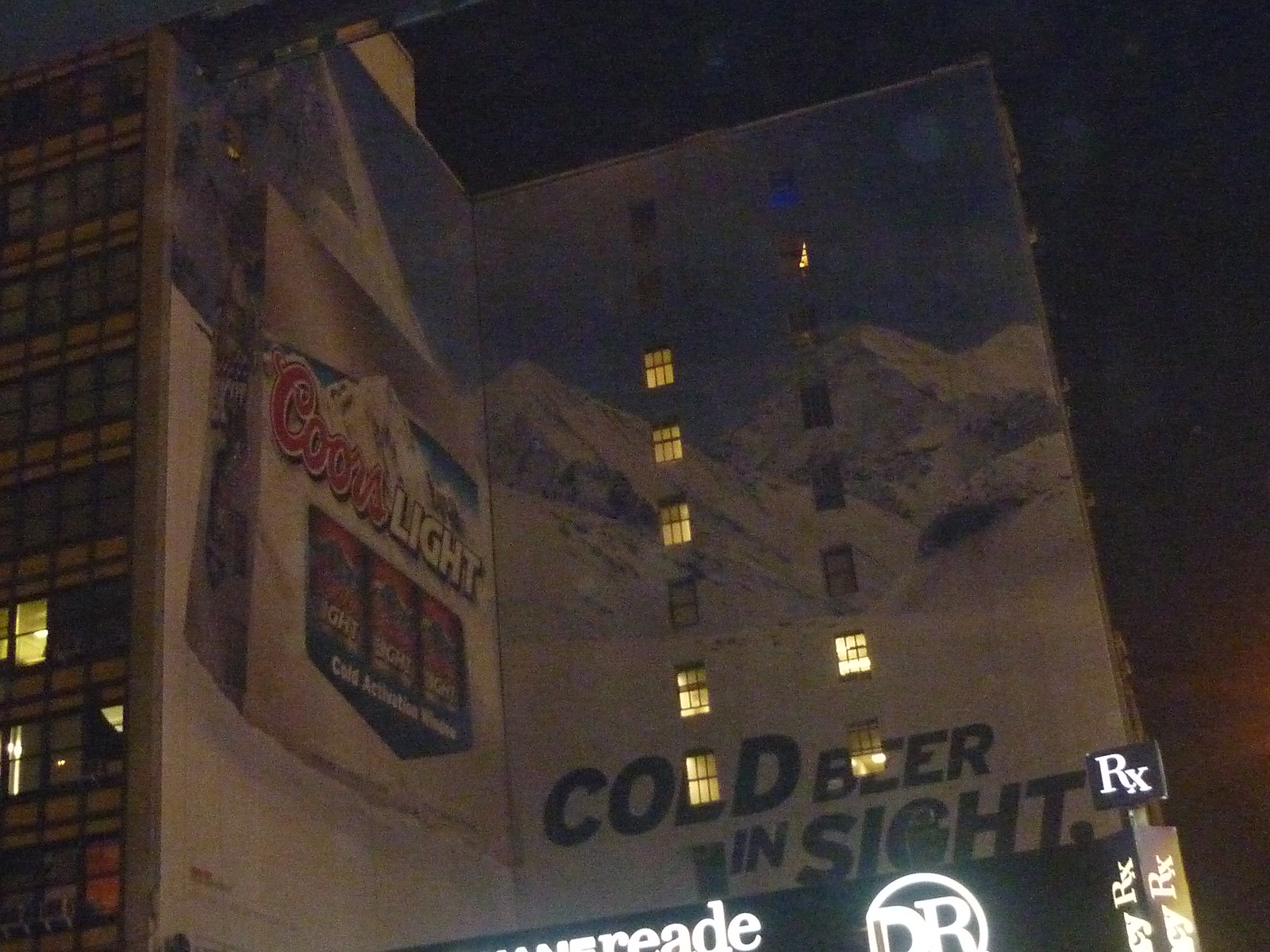This photograph captures a multi-story apartment building against the backdrop of a dark, nighttime sky. The building's staggered windows illuminate the scene with a warm, yellowish glow, though not all of them are lit. Prominently displayed on the side of the building is a billboard advertising Coors Light, subtly illuminated by the ambient light from the windows. On the ground floor, a pharmacy is identifiable by an "RX" symbol and partially obscured but recognizable signage. The words "cold beer in sight" are also painted on a section of the building. Additionally, part of a "Duane Reade" sign, a well-known convenience store and pharmacy chain, is visible but cut off, revealing only the letters "R-E-A-D-E" and a circular "D-R" emblem. The photograph itself appears slightly askew, adding an off-kilter charm to the urban night scene.